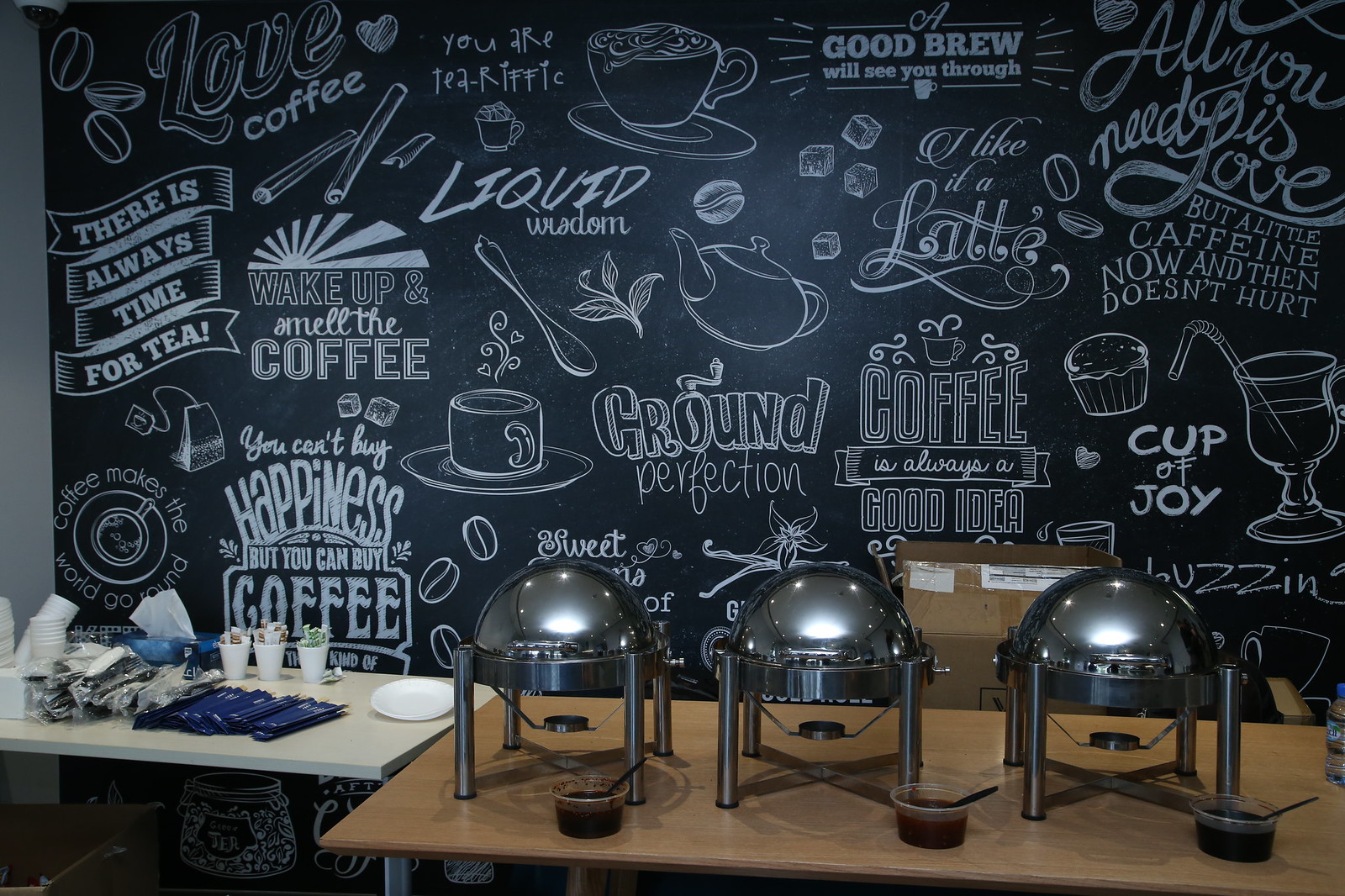This is a color photograph taken in a vibrant coffee shop. Dominating the background is a black wall adorned with whimsical white graphics and text that celebrate coffee culture. The wall features images of coffee beans, sugar cubes, kettles, tea cups, and spoons, alongside phrases like "wake up and smell the coffee," "ground perfection," "cup of joy," and "there is always time for tea," all rendered in various fonts and styles with playful flourishes.

In front of this artistic backdrop, two tables are positioned. On the left is a small white table, neatly arranged with condiments, utensils, and styrofoam cups. To the right stands a larger wooden table that holds three chrome domes on four legs, possibly covering dishes and situated over compartments where candles or burners could be placed for heating. The overall scene is warm and inviting, capturing the essence of a cozy, eclectic coffee shop.